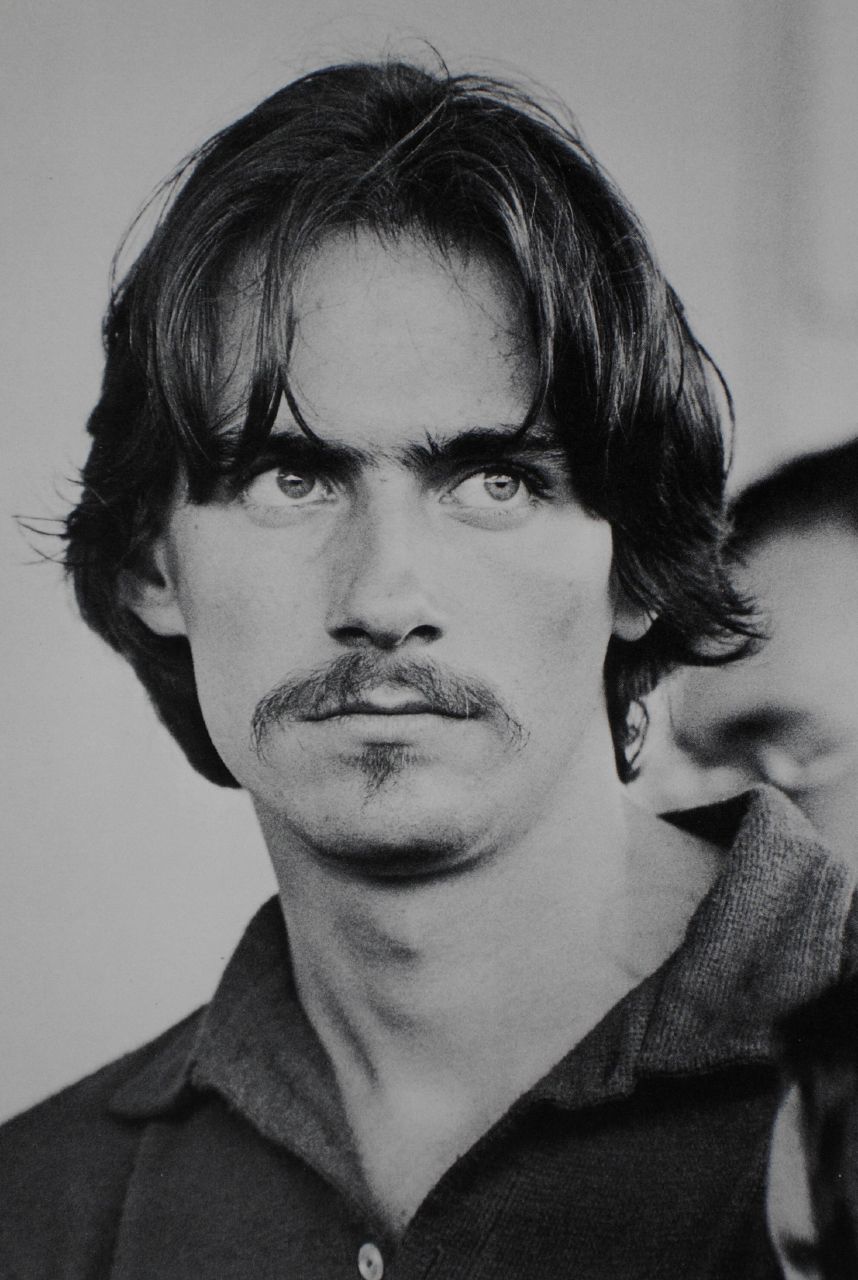This black and white photograph captures a man, likely in his mid-30s, with a serious and somewhat pensive expression as he looks off to his left. His gaze is piercing and he appears focused, perhaps even judgmental. The man sports short, slightly messy black hair that covers most of his ears, and thick, bushy dark eyebrows. His facial hair is minimal, featuring a thin mustache and the beginnings of a goatee. He wears a collared, button-down shirt with the top button visible and the collar resting neatly on his shoulders. The background is plain, emphasizing his contemplative demeanor. This detailed portrait might be a headshot for a movie or TV show, showcasing his intense and striking features.